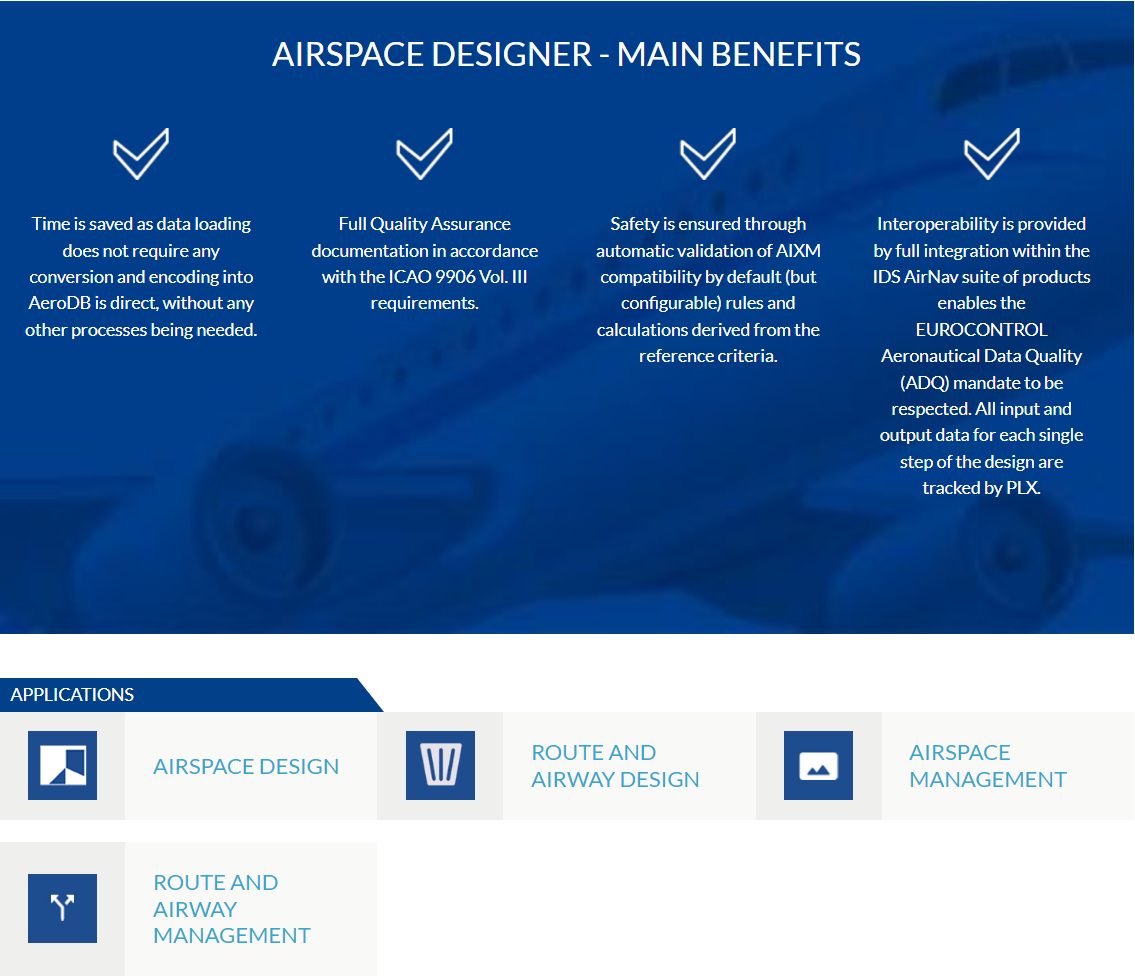This image displays a website with a prominent section showcasing the main benefits of an airspace design service. The overall photo is nearly square and has subtle, undefined borders, suggesting a portrait orientation. At the top is a large, dark blue rectangular banner featuring a watermark-style image of an airplane about to take off towards the right. The banner’s header reads "Airspace Designer Main Benefits" in bold white font.

Below the banner, the content is organized into four columns, each marked with a checkmark icon that has a white outline and transparent blue interior. The first column highlights the benefit "Time is saved as data loading does not require any conversion, and coding into the ARROW DB is direct without any additional processes." The remaining three columns list other benefits, albeit longer descriptions not fully provided here.

Further down, the white background section contains various elements organized into boxes. A blue trapezoid header labeled "Applications" in white font introduces this section. Below this, there are several gray square icons with light gray rectangles beside them, each representing specific applications:

1. A square labeled "Aerospace Design" shaded in light blue.
2. An icon resembling a garbage can, next to the label "Route and Airway Design."
3. A picture icon accompanied by the label "Airspace Management."
4. Arrow symbols going in different directions with the label "Route and Airway Management" in blue.

The overall design and layout suggest this web page is likely part of an advertisement or informational page for an airspace design service or software.